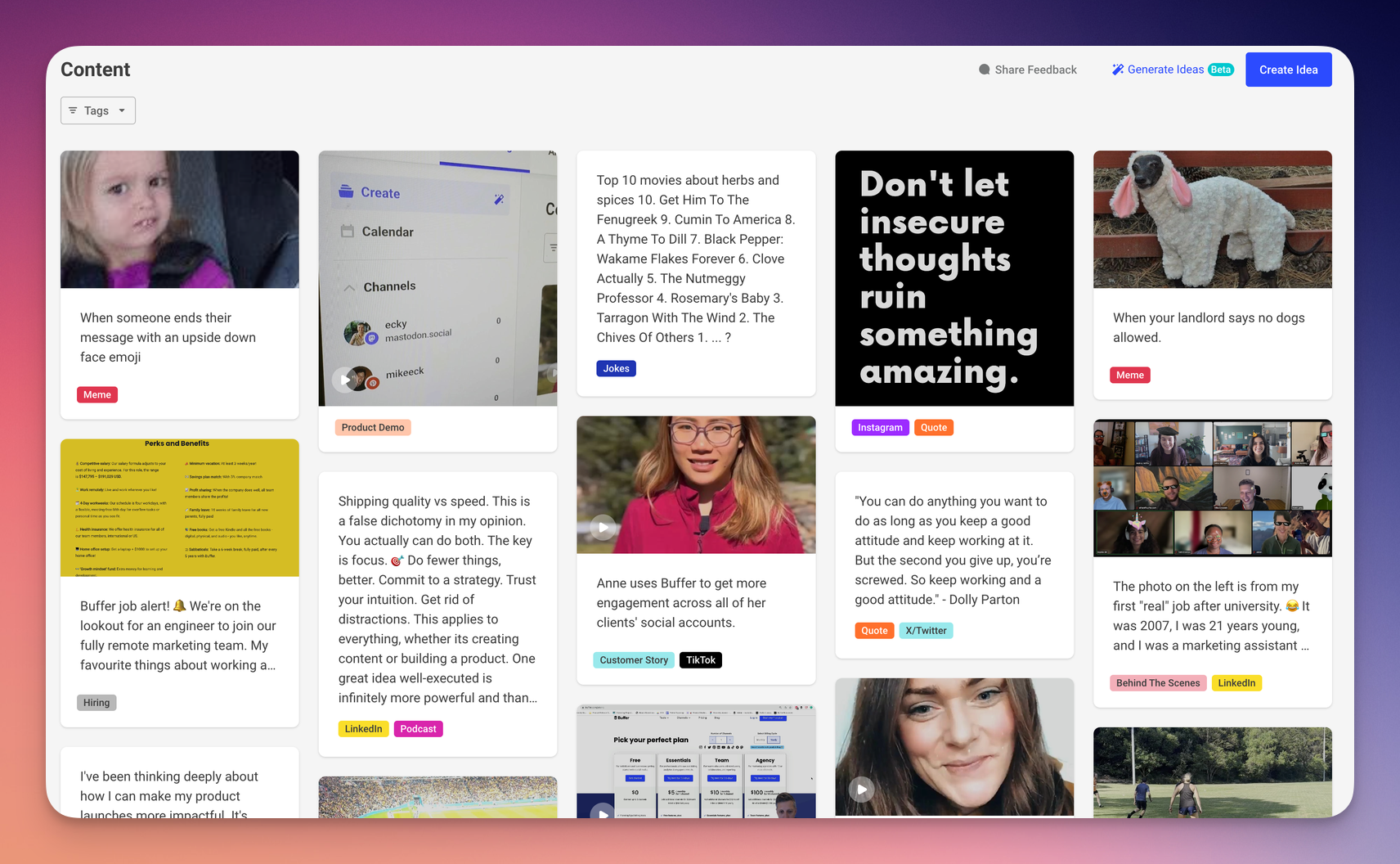In the image, a detailed webpage is displayed. The top left section features a "Contents" header, below which is a filter box labeled with various tags. The main body of the page includes several headlines and captions, one of which features an emoji of an upside-down face, possibly as a meme. Additional segments include a "Product Demo" section, and another labeled "Create Calendar Channels." Separate areas are marked with headings such as "Icky," "Millic," and "Jokes."

A notable section of the page lists "Top 10 Movies About Herbs and Spices," arranged in a countdown format. The entries are:

10. "Get Him to the Greek"
9. "Coming to America"
8. "A Time to Kill"
7. "Black Pepper" (listed twice, suggesting either a repetition or emphasis)
6. "Clove"
5. "The Nutmegging Professor"
4. "Rosemary's Baby"
3. "Tarragon with the Wind"
2. "The Tribes of Palos Verdes"

Adjacent sections also contain miscellaneous details, highlighting a diverse range of topics and features present on the page.